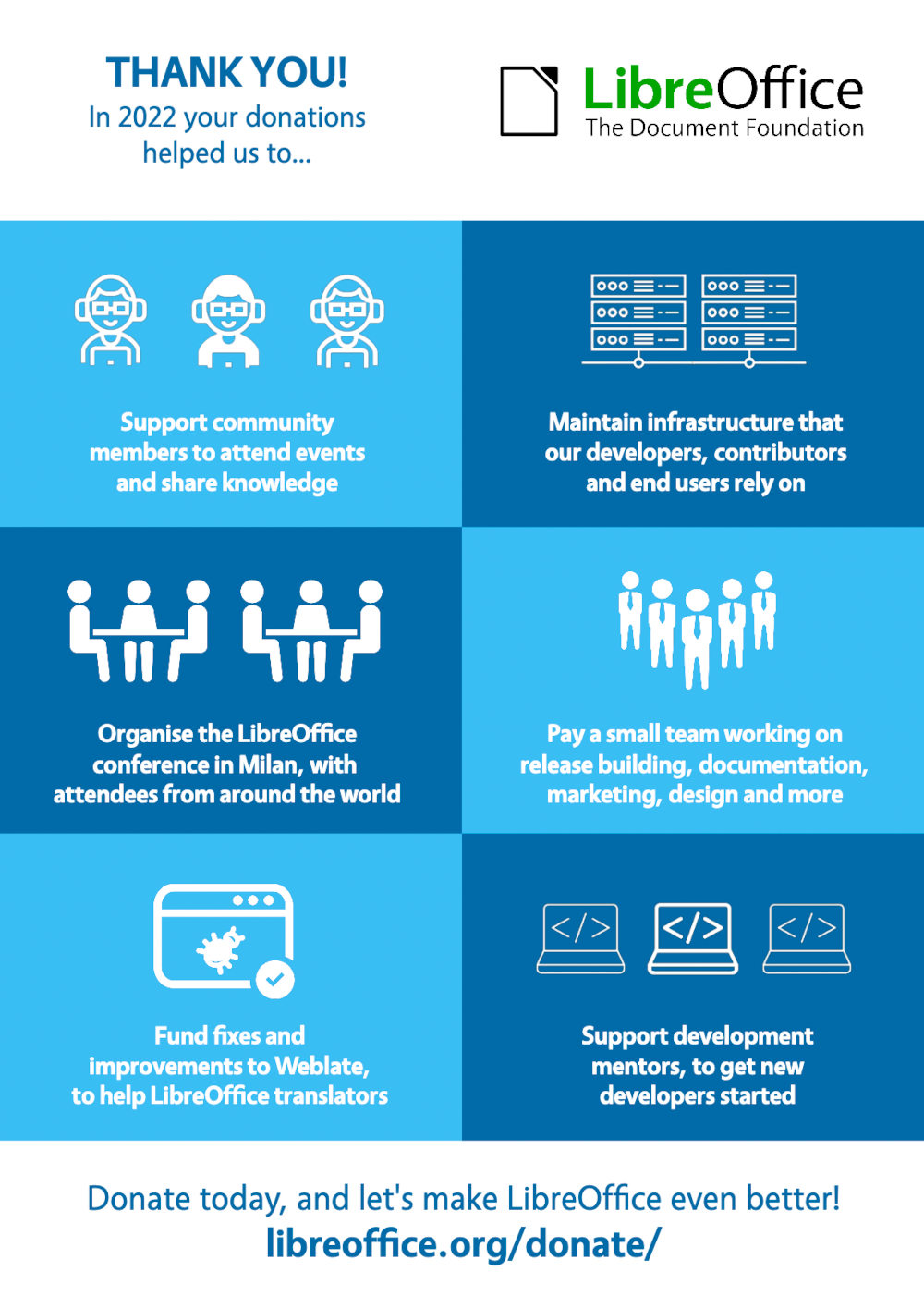This image appears to be a screenshot from a webpage designed to express gratitude to donors. At the top, written in blue letters, it reads: "Thank you. In 2020, your donation helped us to...". Below, a central rectangular field is divided into two columns, each containing three images or infographics in various shades of blue and dark blue.

- **Top-Left Image**: "Support community members to attend events and share knowledge."
- **Middle-Left Image**: "Organize the LibreOffice conference in Milan with attendees from around the world."
- **Bottom-Left Image**: "Fund fixes and improvements to WebLite to help LibreOffice translators."
  
- **Top-Right Image**: "Maintain infrastructure that our developers, contributors, and end users rely on."
- **Middle-Center Image**: "Pay a small team working on release building, documentation, marketing, design, and more."
- **Bottom-Right Image**: "Support development mentors to get new developers started."

Below these infographics, a call-to-action in blue lettering encourages additional donations: "Donate today and let's make LibreOffice even better." This is followed by a link to donate at "libreoffice.org/donate/".

The page likely serves as a blurb, perhaps distributed via email, informing donors about how their contributions have positively impacted various initiatives in the LibreOffice community.